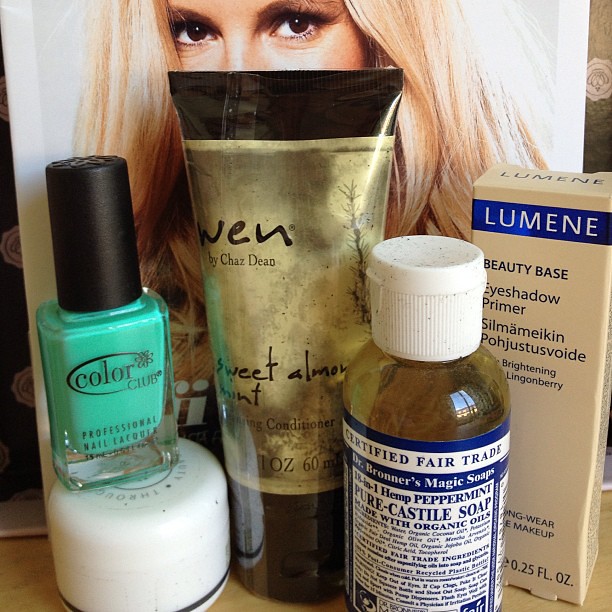This photograph showcases a stylish display of beauty products arranged in front of a promotional card featuring a blonde model with striking eyes and a captivated expression. From left to right, the ensemble includes:

- A small, round white container at the bottom, stack with a bottle of aqua-colored Color Club nail polish featuring a black cap.
- Dominating the center is a black and gold squeeze tube labeled “Wen by Chaz Dean, Sweet Almond Mint, Nourishing Conditioner.”
- In front of this tube stands a bottle with a drip flip white cap, identified as Dr. Bronner's Magic Soap, 18-in-1 Hemp Peppermint Pure Castile Soap, known for containing organic oils and being certified fair trade.
- To the right of this soap is a beige rectangular box with a blue stripe, titled Lumene Beauty Base Eyeshadow Primer.
- All the products are artfully positioned in front of an image of a blonde model, revealing just her engaging brown eyes and shimmering hair, adding a captivating and elegant touch to the display.